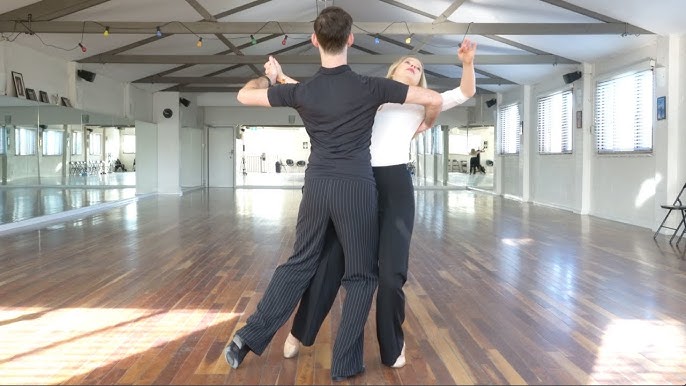In this image, we see a couple engaged in ballroom dancing in a spacious, largely empty studio. The man, who has his back to the camera, is wearing a black t-shirt, black and grey striped pants, and black shoes. He is leading the woman, whose face is visible, and she's dressed in a white t-shirt, black trousers, and silver shoes. The woman appears to be looking up as they move together, with the man's hand placed around her back. The background features high ceilings, wooden floors, mirrors, and windows on both the right and left side. A large door is situated directly behind them, flanked by a few scattered chairs on the right side of the room, emphasizing the expansive nature of the studio.